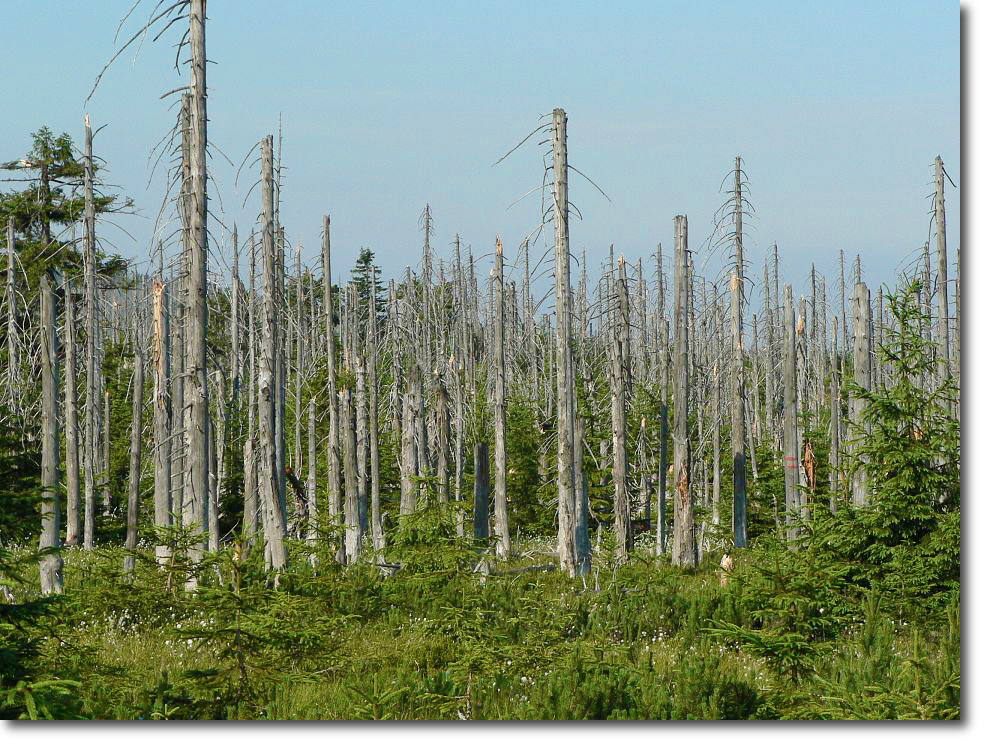The photograph depicts a forest that appears to have endured significant damage, likely from a past fire or a severe windstorm. The central focus is on the tall, denuded pine trees, stripped bare of leaves and pine needles, with skinny, branchless trunks that have a whitish hue. These trees stand rather vertical, reaching up to about two stories high, with their tops snapped off, giving a desolate look. Surrounding these ghostly trunks, the forest floor is lush with tall grass, bushes, and various green vegetation, as well as numerous small pine seedlings and five-foot tall trees indicating ongoing regrowth. In the background, there are some fully intact trees with branches and leaves, contrasted against the bluish-gray sky overhead, creating a somber yet resilient scene.